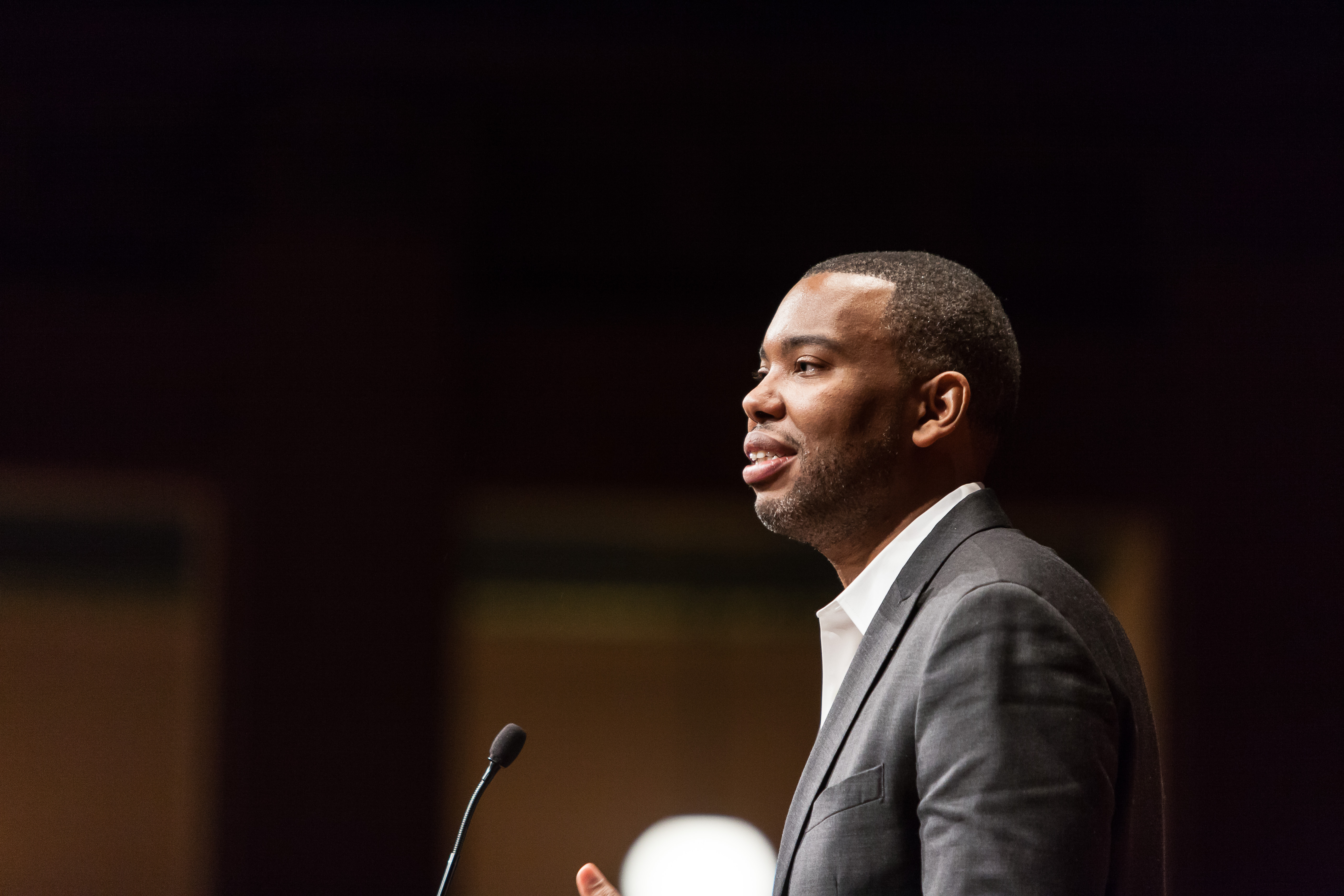The photograph features a young African-American gentleman, estimated to be between 25 and 30 years old, captured from a profile-type angle while he is speaking into a thin, podium-style microphone. He has very short hair and a slight dusting of facial hair, including a mustache and a beard. The man is dressed in a gray suit jacket paired with a white button-down long sleeve shirt, but he does not wear a tie. His right hand, with the thumb visible, is positioned just below the microphone. The background is predominantly dark, with hints of yellowish-brown, suggesting window areas, and there is a circle of light visible just behind his thumb. The image focuses solely on the man, with the background details being largely unremarkable.